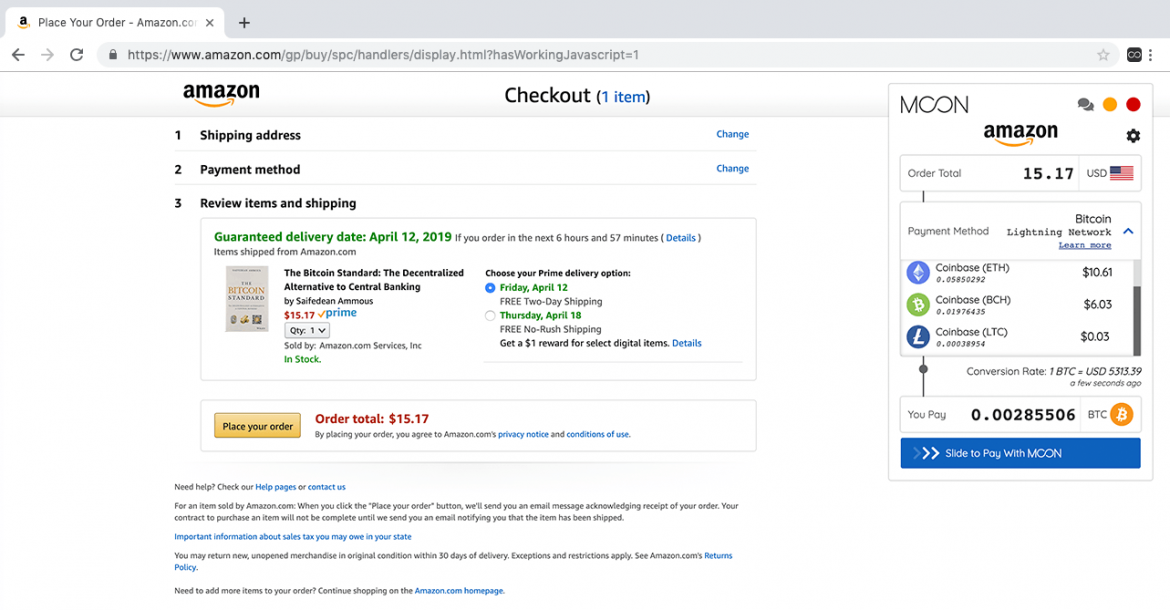The image features a detailed checkout screen from Amazon's website, prominently displayed on the top left tab as "Place Your Order - Amazon.com." At the top center of the screen is the Amazon logo, beneath which reads "Check Out 1 Item," with the quantity "1 Item" highlighted in blue. 

1. **Shipping Information:**
   - **Shipping Address**: The section is labeled as 'number one' with a separate blue button labeled 'Change.'
   
2. **Payment Method:**
   - **Payment Method**: Listed as 'number two' with a change button situated on the right side.

3. **Review Item and Shipping:**
   - **Review Item and Shipping**: Marked as 'number three,' it includes information about the guaranteed delivery date, stated in green as "Guaranteed delivery date: April 12, 2019, if you order in the next 6 hours and 37 minutes" and notes that items are shipped from Amazon.com.
   
The specific item listed for purchase is "The Bitcoin Standard: The Decentralized Alternative to Central Banking" by Saifedean Ammous, priced at $15.17, with a quantity of 1 and confirmed as "In Stock" — the stock status also highlighted in green.

**Delivery Options:**
- Options include free Prime delivery on Friday, April 12, with this option being highlighted in green. Another option listed is No-Rush Shipping with a delivery date of April 18.

At the bottom, the yellow "Place Your Order" button is prominently displayed, along with the order total of $15.17, which is noted in red text. The payment methods available are diverse, including Bitcoin via the Lightning Network, Coinbase Ethereum ($10.61), Coinbase BCH ($6.03), and Coinbase LTC ($0.03), with conversion rates listed as 1 Bitcoin equaling $5,039.10 USD. The total Bitcoin amount required is 0.00285506 BTC. The bottom of the image features a blue button labeled "Slide to pay with Moon" for completing the Bitcoin payment.

This elaborate checkout screen captures the variety of modern payment options available and the comprehensive details provided by Amazon for placing an order.